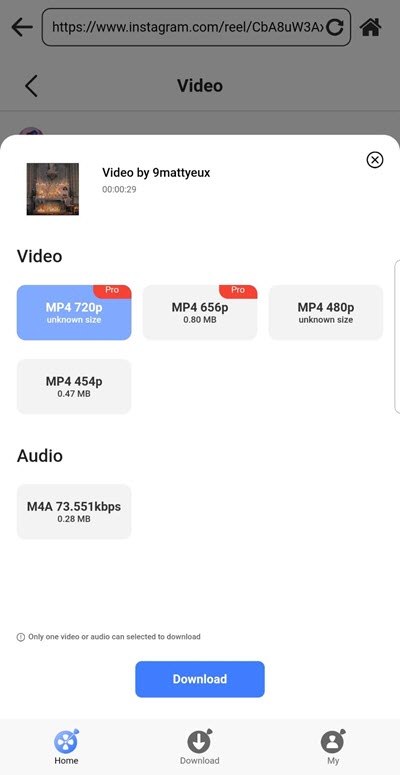The image appears to be a screenshot taken from someone's phone, displaying a web application with an Instagram interface. The upper part of the image shows a navigation bar with the Instagram website URL and a home icon to the right. Beneath this bar, there is a heading that reads "video."

At the bottom center of the screen, there is a pop-up box with a white background. This pop-up indicates "video by 9mattieux" and includes a square thumbnail to the left, which features a gray background and the faint outline of a person who might be wearing a tan vest. To the right of the center text, there is a circular button labeled "XL."

Below this section, the pop-up is divided into two categories: "Video" and "Audio." In the "Video" section, there are four rectangles, with the top left one highlighted in blue, labeled "MP4 720p." In the "Audio" section, a single rectangle displays "M4A 73.551 KBPS."

At the very bottom in the middle of the pop-up, there is a prominent blue download button. The footer of the screen has a gray background and three icons. The "Home" icon, which resembles four arrows pointing outward, is followed by the "Download" icon featuring a downward arrow, and lastly, the "My" icon, which resembles a generic profile or account icon.